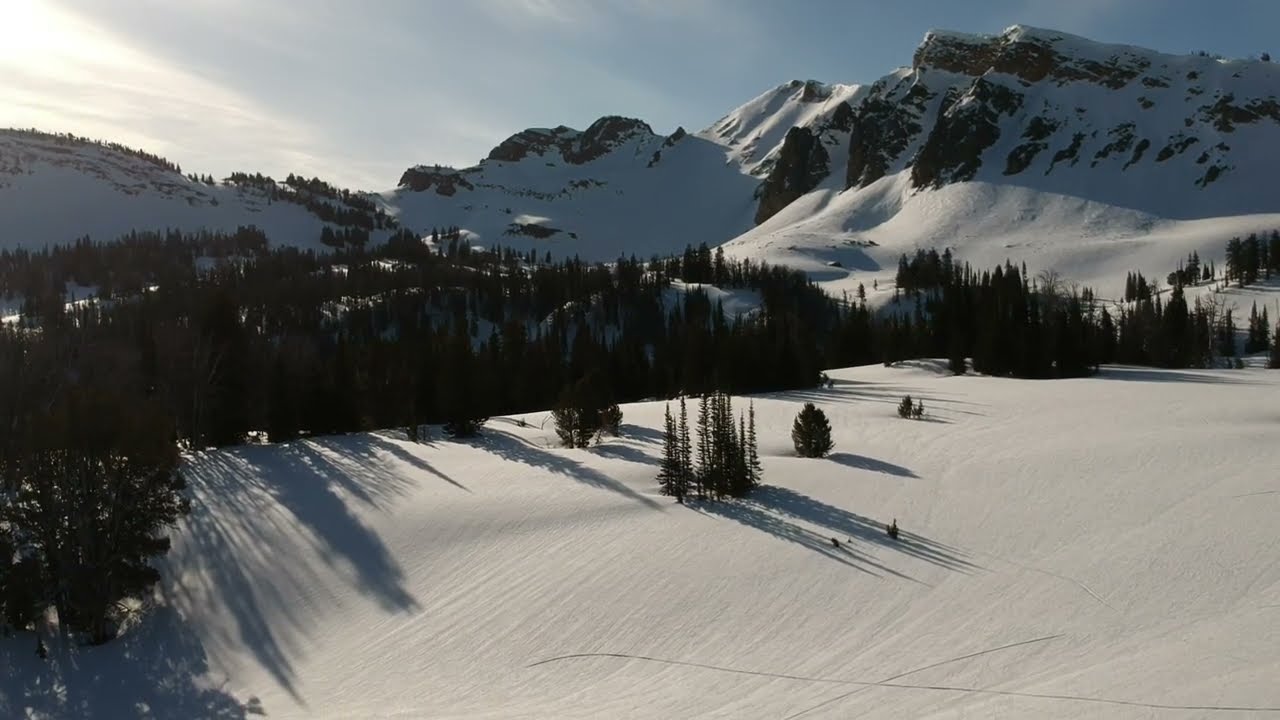The photograph captures a breathtaking snow-covered mountain scene taken from a high vantage point, possibly from a drone or a ski lift. The foreground showcases a wide, open field blanketed in pristine snow, creating a striking contrast with the dense clusters of pine trees that stretch across the middle of the frame. The pine trees are dark and densely packed, casting long shadows onto the snow due to the sunlight breaking through the grayish-blue sky, which is laced with wispy clouds. The subtle paths crisscrossing the snow suggest it may be part of a beginner section of a ski slope. In the background, imposing mountaintops draped in snow rise majestically, with rugged rocks peeking through the white. The scene is reminiscent of a tranquil, unspoiled ski resort landscape, embodying the serene beauty of a winter wonderland.